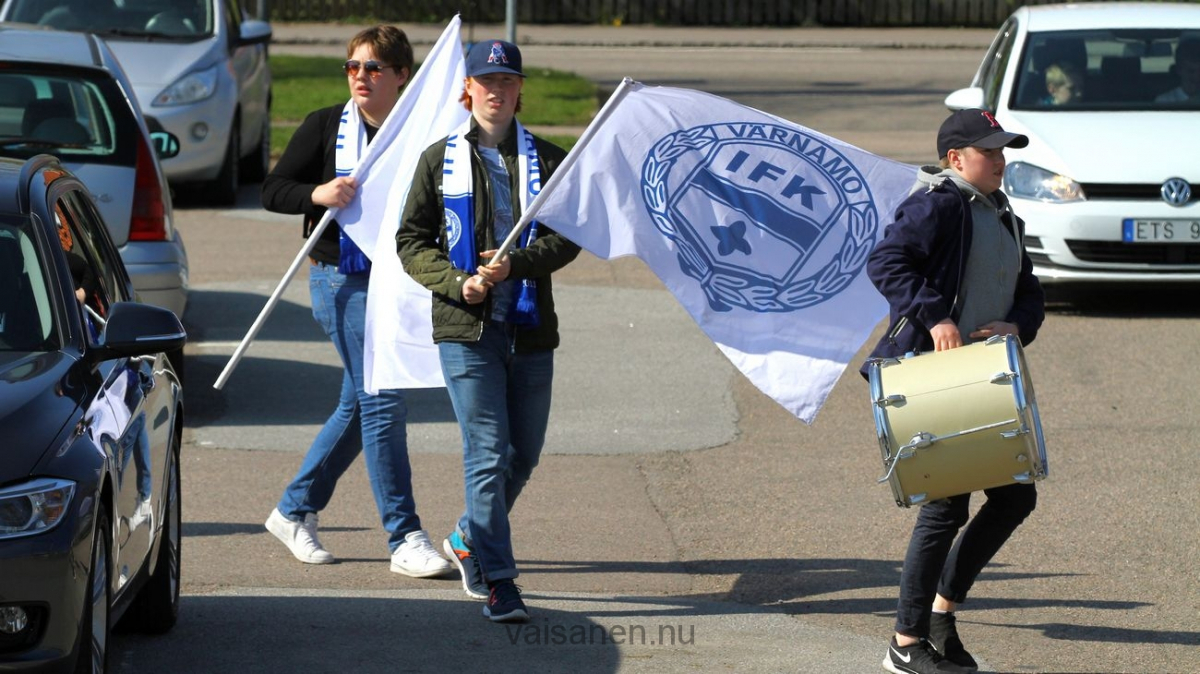In this image, a residential street, potentially a parking lot near a school, is depicted in broad daylight under a clear, sunny sky. On the left side of the image, a series of parked cars is visible, including a prominent white Volkswagen with license plate beginning ETS. The car harbors a man in the driver’s seat and a younger person with blonde hair in the passenger seat. In the background, additional cars can be seen.

The focal point of the image centers on three individuals walking across the street, likely heading towards an event, possibly a parade or sporting event. Leading the group is a young boy dressed in a dark baseball cap, a blue jacket, black jeans, and black sneakers. He carries a yellow drum. Behind him, a person dressed in blue jeans, blue sneakers, and a green jacket walks, holding a white flag. This individual also has a black baseball cap and a scarf, suggesting a fall setting. Lastly, a third person, wearing a black shirt, blue jeans, and white sneakers, follows them, carrying a flag that bears the text "Varnamo IFK" and "Veysanen.nu." The array of colors in the image includes white, blue, silver, yellow, red, and black, adding to the lively and detailed scene.